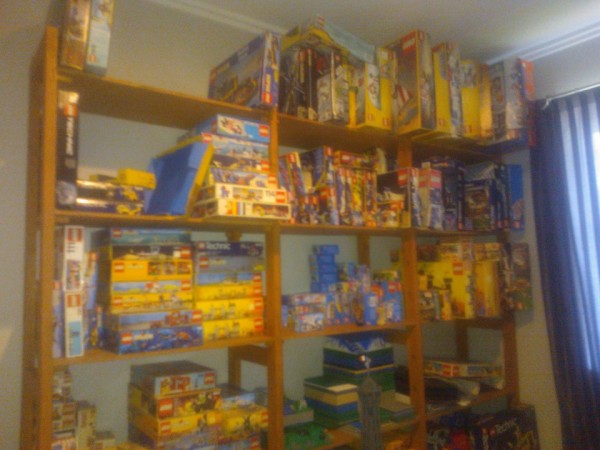The image depicts a room within a flat, characterized by light green walls and a white ceiling. Dominating the scene is a large brown wooden bookshelf, which is organized into three sections with a total of 15 dividers. To the right of the bookshelf, a blue curtain covers a window, allowing filtered light to seep through.

The bookshelf is primarily filled with various Lego set boxes, which are mostly yellow, with some blue and green boxes interspersed. These boxes are arranged in a somewhat color-coordinated fashion. The top right section of the bookshelf is completely stacked with these Lego boxes, arranged vertically, while the other sections have a mix of horizontal and vertical placements with gaps in between some boxes. Notably, the tall top left shelf section contains only three Lego boxes, with two on one side and one on the other, contrasting with the densely packed nature of the rest of the shelves.